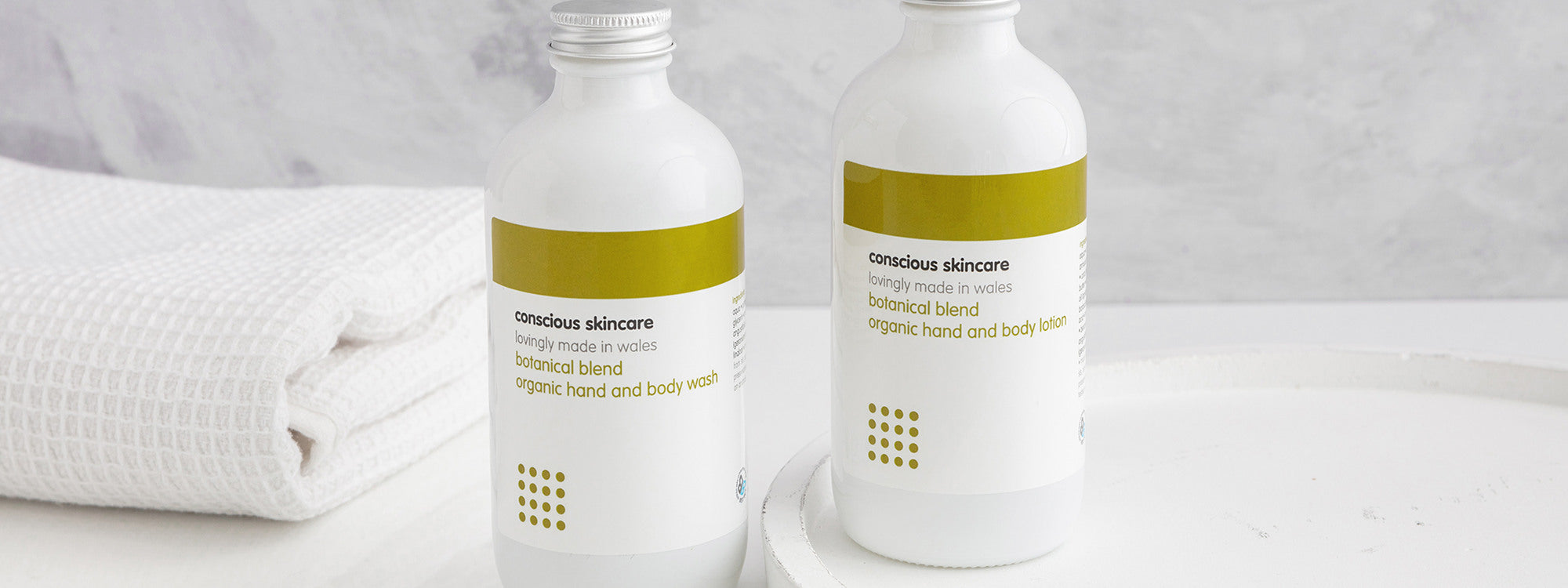This detailed landscape photograph, seemingly an advertisement, showcases a luxurious display of Conscious Skin Care products. Centered on a pristine, white reflective marble countertop, two identical white bottles with silver screw-on caps are presented. These cylindrical bottles taper gracefully at the neck, adorned with clean, white labels accentuated by a sophisticated gold band. The text on the labels, though partly blurred, prominently reads in black, "Conscious Skin Care," and below it, in the same green hue as the gold band, "Lovingly Made in Wales," "Botanical Blend," and "Organic Hand and Body Wash." To the left of the frame, an immaculately folded waffle-patterned towel adds a touch of domestic comfort. Behind the bottles, a striking backdrop of light grey marble with intricate striations enhances the scene's elegance. One of the bottles is elevated on a distinct white, rounded platform, possibly a tray or pedestal, featuring subtle grey marks indicative of wear. This platform is partially cut off at the image's bottom edge, suggesting a dynamic visual composition. The meticulous alignment of these elements conveys a serene and sophisticated bathroom or skincare setting.